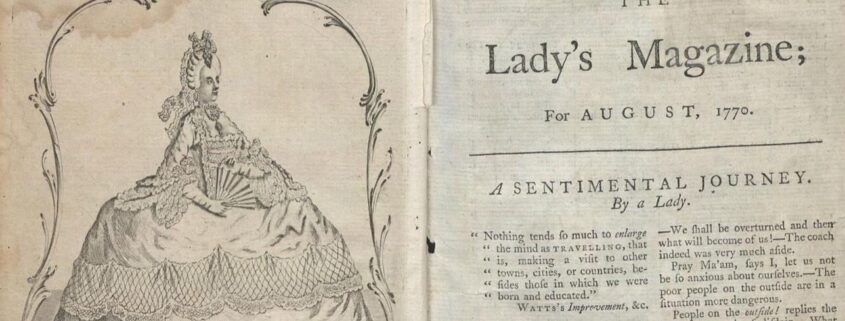This is a photograph of a page from "The Ladies' Magazine" for August 1770, featuring an article titled "A Sentimental Journey by a Lady." The left side of the page showcases an intricate black-and-white illustration of a woman dressed in extremely elaborate Victorian-era clothing, including a massively wide, ornate dress and a detailed, either styled or adorned, wig or headdress. She holds a fan in one hand and is framed by decorative scrollwork and filigree patterns that add to the image's ornate quality. The illustration, although a line drawing, provides enough detail to convey the scene's grandeur and historical context. On the right-hand side of the spread, aged and stained, some text is visible, starting with, "Nothing tends so much to enlarge the mind as traveling," and continues to describe the perils of a coach journey, emphasizing consideration for others' safety. The text, coupled with the detailed illustration, gives a glimpse into the themes and aesthetic sensibilities of 18th-century lady's magazines.